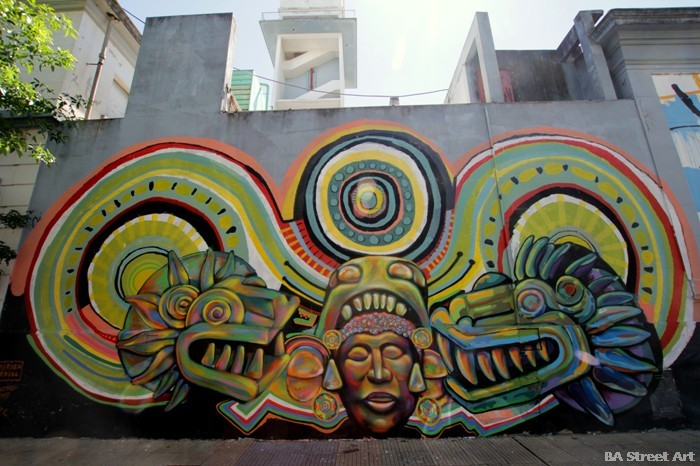Captured from a distance, the image showcases a vibrant and large mural, painted on a substantial stucco wall that's part of a residential building complex. The mural, bursting with bright neon colors including yellow, green, blue, pink, and orange, features a detailed figure representing an Aztec or Mayan god or priest. This central figure is adorned with an elaborate headdress that intertwines with two mythical creatures, possibly lions or dogs, emanating from both sides of the priest. These creatures have jagged teeth, with one embodying daylight and the other representing night. The mural's background is filled with an intricate, abstract circular design suggestive of sun worship, common in Mesoamerican art. Notably, in the bottom right-hand corner of the mural, the text "B.A. Street Art" is visible, indicating the artwork’s watermark. The photograph captures the mural under clear sunny skies, although the image is slightly out of focus.